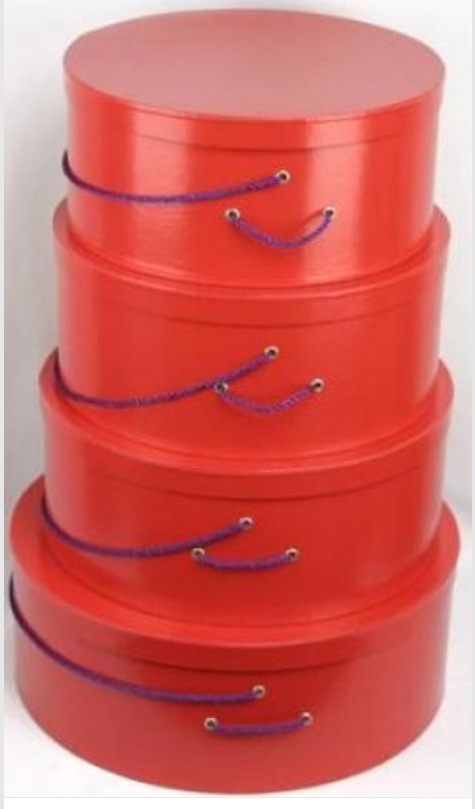This photograph features four graduated, circular containers, each with a glossy orange finish and matching lids. The containers are stacked neatly on top of each other, with each box slightly smaller in diameter than the one below it. The difference in size between the largest box at the bottom and the smallest at the top is approximately three to four inches. Each box has brass grommets through which a short purple rope handle is threaded, lined up uniformly so that the longer handles are positioned on the left side of the stack. The image is set against a plain white cream background, enhancing the vibrant colors and reflective surface of the containers. The handles resemble strong purple shoelaces, providing both a decorative and functional aspect to the design. The reflective quality of the boxes' surface suggests a sleek, polished finish, with beams of light particularly visible on the top container.